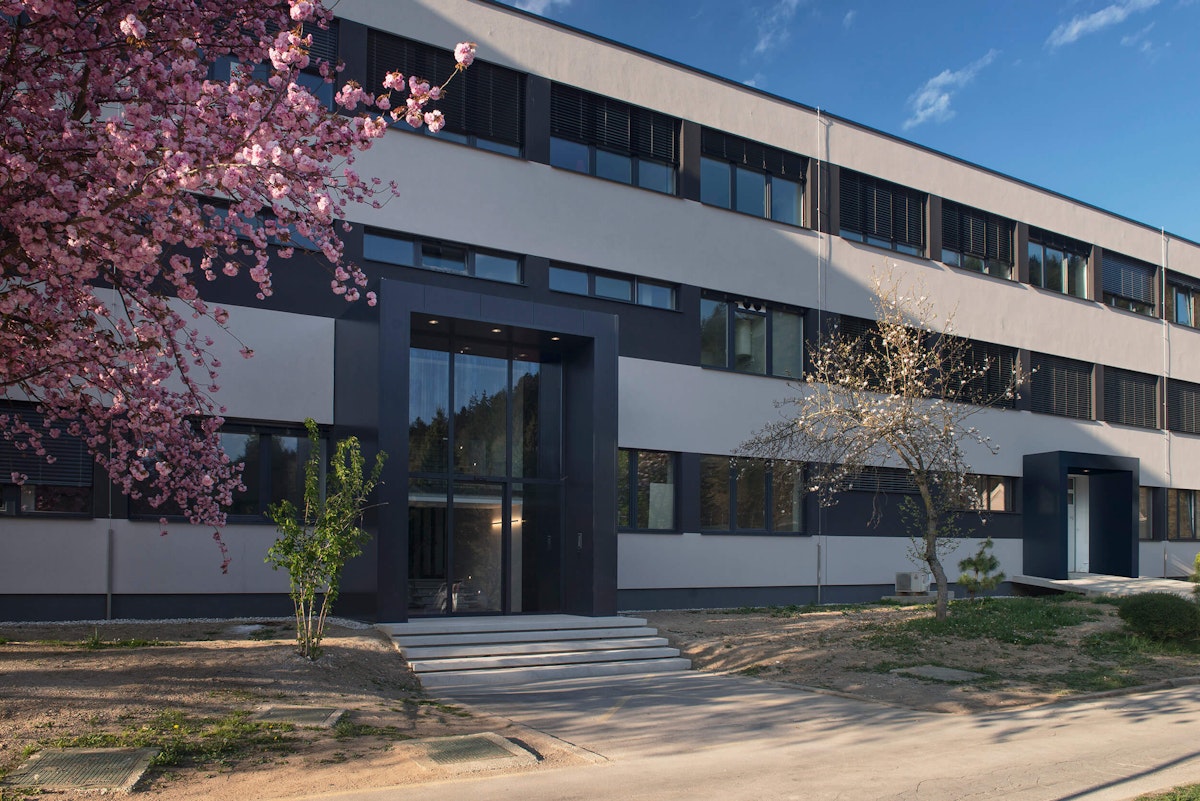The image depicts a three-story building, which could be either an apartment complex or a business facility, featuring a large, prominent entrance with steps leading up to it at the front and center of the structure. The building is predominantly white, accented with dark blue or black around the numerous windows and outlining the main door. To the right of the frame, there's a secondary, smaller entrance without stairs. The foreground showcases a bare lawn flanking the walkway to the central entrance. Notably, there's a shorter tree with white flowers, positioned closer to the right side of the building, reaching the second floor, and a taller tree on the left side, possibly a cherry blossom, extending up to the third floor or higher, adorned with pink flowers. The overall scene is devoid of people.